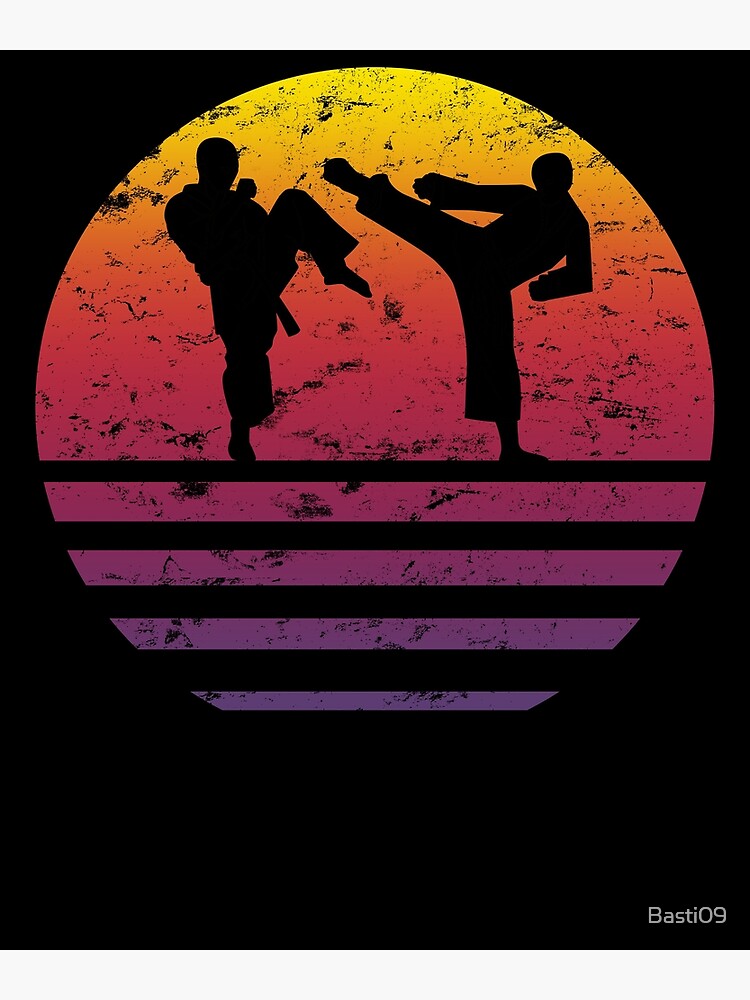The image is a vertically rectangular digital art piece with a black background and no border. Dominating the composition is a textured circle resembling a sunset, with a gradient that transitions from yellow at the top to orange, pink, and finally purple or blue at the bottom. Within this circle, two martial artists in silhouette, engaged in karate moves with their legs raised in an attack posture, are the focal point. The scene is further enriched by rough black ink textures that give the sunset a more tactile and dynamic feel. Below the silhouettes, vertical black lines extend from the center of the circle to its bottom, adding depth and interest to the image. In the very lower right-hand corner, the text "BASTI09" is inscribed in white.